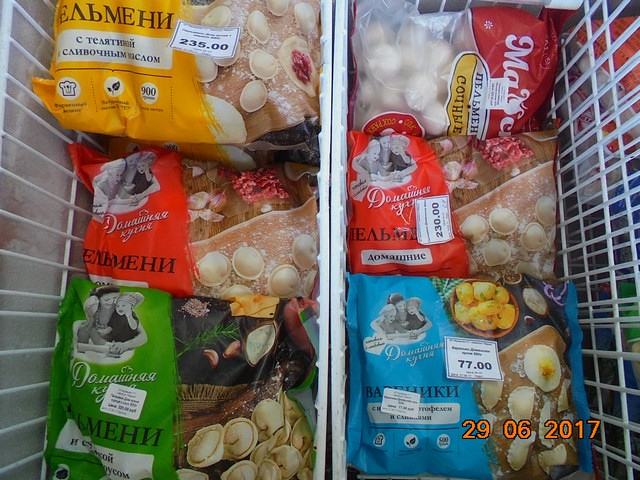This photograph captures a downward view into the nearly empty freezer bins of a store, likely taken on June 29, 2017. The bins, lined with white refrigerator racks, contain six colorful packages of what appear to be frozen pasta, such as ravioli or gnocchi. These packages are arranged in three rows with two columns each. The bags showcase a variety of colors—yellow, red, green, and blue—and prices like 235.00 and 230.00 are visible on some of them, though the text is in a foreign language, possibly Russian. One package displays an image suggesting they are made with potatoes, adding a specific detail to their content. The partial inclusion of a third bin hints at the potential for more of the same product.